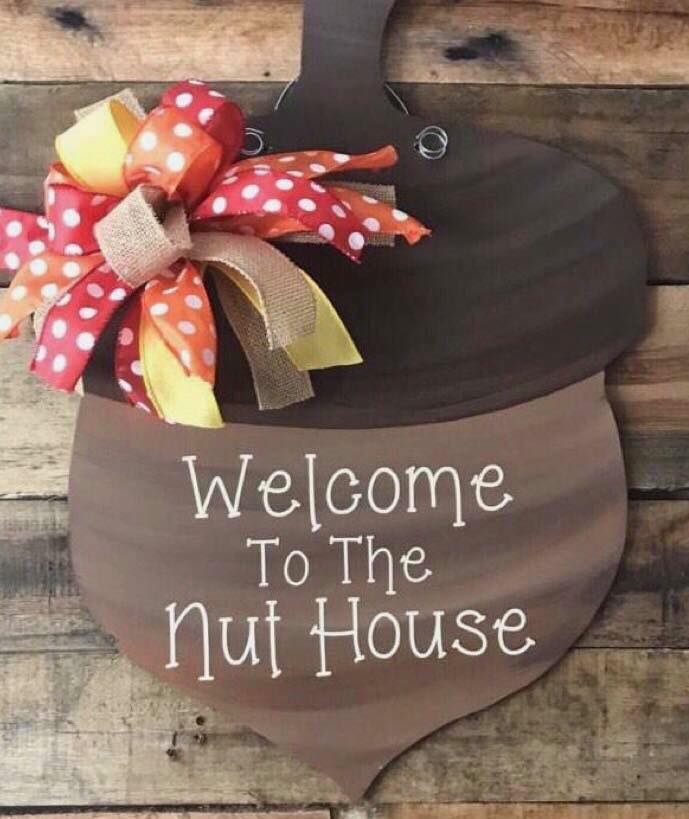This image shows a handmade, kitschy sign in the shape of an acorn, positioned against a rustic wooden background, likely a wood-paneled wall or the side of a barn. The acorn, crafted from a single flat piece of board, is meticulously painted to mimic the natural colors and textures of an actual acorn. The top half, representing the acorn's cap and stem, is painted a dark brown with brush strokes that curve to follow the cap's natural arch. The bottom half is painted in a lighter brown with similar curved strokes to mirror the acorn's shape. A playful, thin-fonted white text across the bottom part of the acorn reads "Welcome to the Nut House." Adorning the top left corner is a decorative bow made of various ribbons—orange, red, yellow, and beige canvas—with the orange and red ribbons featuring white polka dots. This charming, DIY decorative piece exudes a warm, welcoming aura, suggesting it's designed to greet visitors at the entrance of a home nicknamed "the nut house."